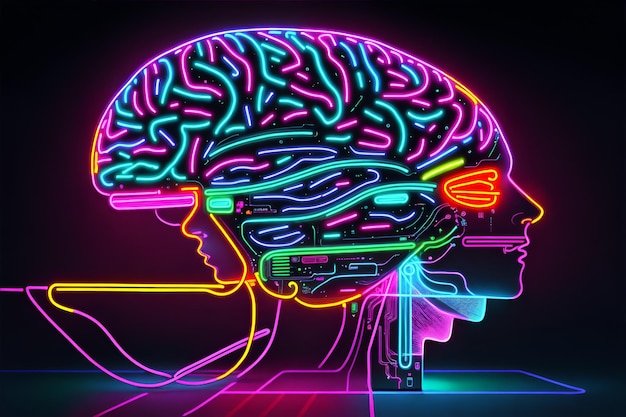This striking piece of neon-style abstract artwork portrays a highly stylized and artistic rendering of human heads and an oversized brain. Set against a solid black background, the image features two profiles merged together, each head outlined and detailed with vibrant, glowing neon lines in colors such as pink, purple, cyan, green, yellow, and orange. The heads, one larger and facing right with a distinctively human-like eye, nose, and mouth, and the other facing opposite with a defined nose and mouth but without eyes, are connected at the brain, which sprawls above them in an intricate mesh of neon strips primarily in pink and light blue. Extending from the bottom of the heads, glowing lines cascade downwards and converge on a surface illuminated with red and cyan hues. The entire composition gives a futuristic, fantasy-like impression, merging elements of human anatomy with imaginative neon artistry.